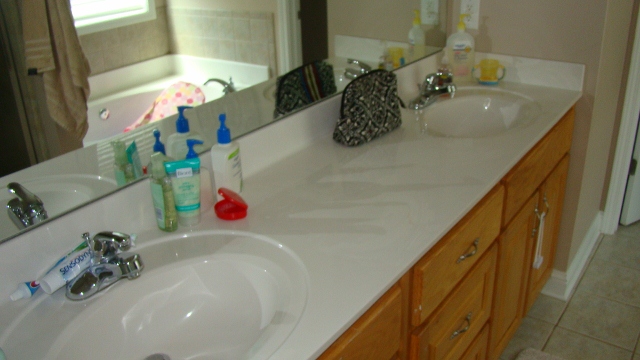A photograph captures a well-utilized double vanity bathroom setup. The foreground features a countertop with two distinct sink areas. In the lower left corner, the first sink is accompanied by grooming essentials: a tube of Sensodyne toothpaste placed just behind it, and a tube of Crest toothpaste nestled further back. Adjacent to this sink, directly in front of a towering mirror, a small collection of bottles including soaps and lotions adds a touch of everyday functionality. Among these is a red plastic container for a mouth guard or retainer, its lid casually flipped open.

Progressing towards the upper right-hand corner of the image, a black and white makeup or travel bag rest atop the counter, reflecting convenience and a touch of personal style. Here, the second sink marks the end of the double vanity. In the corner, where the countertop meets the wall, additional personal care items are arranged, including another soap bottle and what resembles a child’s sippy cup, possibly indicating infant baby soap.

The mirror offers a seamless reflection of the bathroom’s opposing side, revealing a bathtub accompanied by a tan shower curtain and a light brown towel hanging nearby. The overall scene evokes a sense of a functional and lively family bathroom.